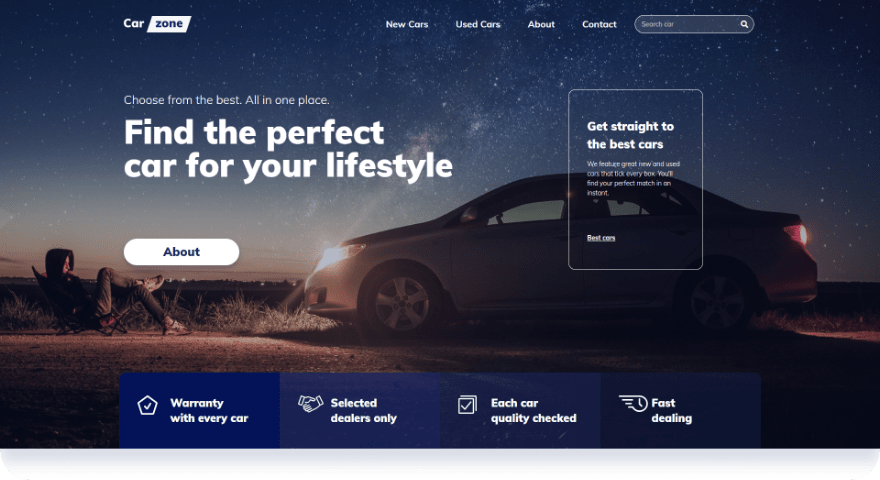Under the category of websites, the top left corner prominently displays "Car Zone". To its right, there are navigation options labeled "New Cars", "Used Cars", "About", and "Contact". Adjacent to these is a search bar featuring a magnifying glass icon. Below, a slogan reads, "Choose from the best all in one place. Find the perfect car for your lifestyle." Further down, a white bar is marked "About" and a white box declares, "Get straight to the best cars."

At the bottom, several features are highlighted: "Warranty with every car," "Selected dealers only," "Each car quality checked," and "Fast dealing."

The entire layout is set against a stunning background image of a deep blue, starry sky with countless stars illuminating the scene. In the distance, majestic mountains can be seen. In the foreground, a man--dressed in a hoodie, jeans, and sneakers--is sitting in a camp chair on the dirt with patches of grass around, creating a very rural atmosphere. He is positioned in front of a light gray or silver four-door sedan, which has its headlights turned on, casting light on him. The car's tires and rims are clearly visible despite the darkness.